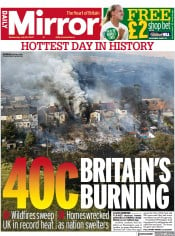This image is a magazine cover from the Daily Mirror. The background of the cover is predominantly red, featuring bold white text for the magazine's title. At the top, two headline articles capture immediate attention. The first headline reads "Hottest Day in History" in bright red letters against a stark white bar, indicating a record-breaking temperature of 40 degrees Celsius. The subheading dramatically states "Britain is burning."

A central, albeit slightly blurry, image occupies the cover's middle. It depicts a town engulfed in flames, emphasizing the catastrophic conditions caused by widespread wildfires. The accompanying text describes the scene as "Wilderness, UK in record heat" and notes the devastating impact with "Homes wrecked as nations swept theirs."

Towards the bottom of the cover, there's a smaller article, likely giving more details on the ongoing crisis. Additionally, a green square positioned to the right side of the cover advertises a free offer with the text "Shop better." A person wearing a white shirt is also visible, possibly related to the promotional content.

Overall, the cover uses contrasting colors—red for urgency, white for clarity, and green for promotional attractiveness—to convey a sense of immediate crisis and pressing news.